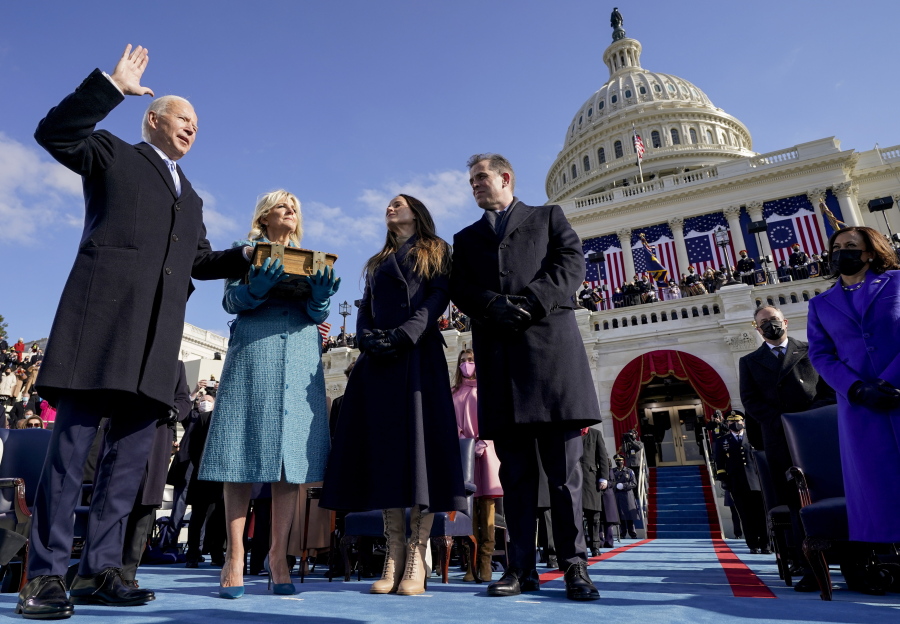This photograph captures the historic inaugural swearing-in ceremony of President Joe Biden at the U.S. Capitol. In the center, President Biden, wearing a long black coat, dark blue pants, and black shoes, stands with his left hand placed on a Bible held by his wife, Jill Biden, and his right hand raised in oath. Jill Biden is elegantly dressed in a blue coat, gloves, and shoes. To the right of Jill Biden stands Vice President Kamala Harris, attired in a long black coat and tan boots, accompanied by her husband, who is dressed entirely in black, including a black coat, pants, gloves, and shoes.

The scene is set against the backdrop of the Capitol building, with its iconic white dome prominently visible. American flags adorn the building, while the sky above is clear blue with a few white, puffy clouds. On the ground, a blue carpet with red stripes leading up the stairs marks the ceremonial pathway. Numerous onlookers are present, both on the ground and on a balcony above, some seated and others standing. The atmosphere is formal, with everyone dressed in winter clothing, highlighting the solemnity and importance of the occasion.